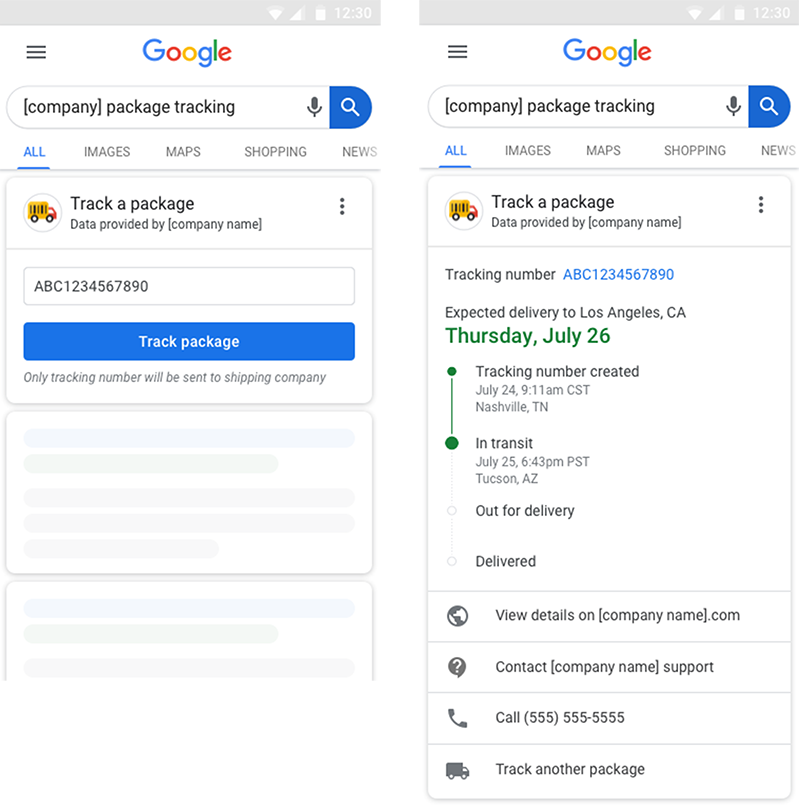In the image, there are two smartphone screens displayed side by side, both showing a Google search results page. The time on both phones is 12:30, and in the top right corner, there are icons indicating Wi-Fi connectivity, signal strength, and battery life. 

The Google logo is prominently featured at the top of the screen, with each letter in a different color: the 'G' in blue, the first 'O' in red, the second 'O' in yellow, the 'L' in green, and the 'E' in red. Below the logo is a search bar with the text "company, package tracking". Beneath the search bar, there are various tab options such as "All," "Images," "Maps," "Shopping," and "News," with the "All" tab being highlighted.

On the left screen, the page displays a section titled "Check a Package" with data provided by a company. There's a blue button labeled "Track Package". Below this button, there is a note stating "Only the tracking number will be sent to the shipping company."

On the right screen, the page is nearly identical but includes additional tracking information. It states "Express delivery to Los Angeles, CA," with the date "26 July" written in green. It also provides a timeline: a tracking number was created on "July 24, 11:11 a.m. CST in Nashville, TN"; the package was "In Transit on July 25, 6:43 PST in Taxi, AZ"; and the status is currently "Out for Delivery." 

The bottom of both screens includes the text "View details on companyname.com," alongside a "Contact" section with "Company Name" and a phone number "Call 55555," followed by an option to "Check another package."